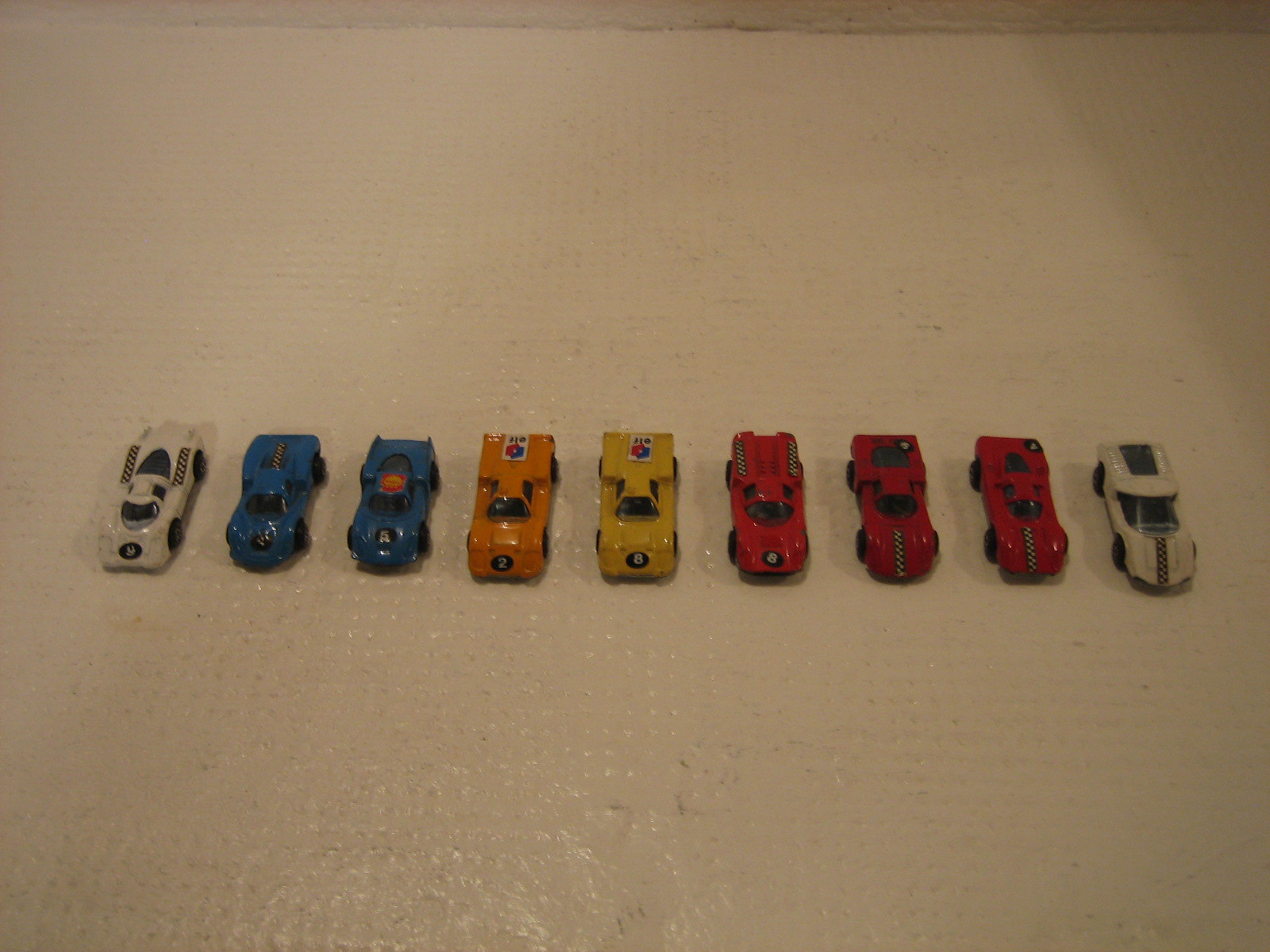The colour photograph, taken under yellowish indoor lighting, depicts a row of scale model cars lined up horizontally from left to right. The image quality is low, likely captured with a low-quality smartphone or an older digital camera, resulting in a less sharp resolution and muted colours. The cars, resembling Hot Wheels or Matchbox-style toys, are positioned with their fronts facing the viewer, spaced about an inch apart, and set against a surface with slight texturing that reflects light subtly. Starting from the left, the first car is black with a white number '9' on the hood. Following are two blue cars with unreadable numbers in black circles on their hoods, a vivid orange car marked with a white '2' in a black circle, a yellow car with a white '8' in a black circle, a red car also with a white '8' in a black circle, two red cars with checkered racing stripes on their hoods, and finally, a white car adorned with a black and white checkered flag stripe. The overall scene is framed by what appears to be an off-white textured surface, possibly a rug or a mat, under moderate lighting that adds a slight reflective quality to the image, especially at the front.